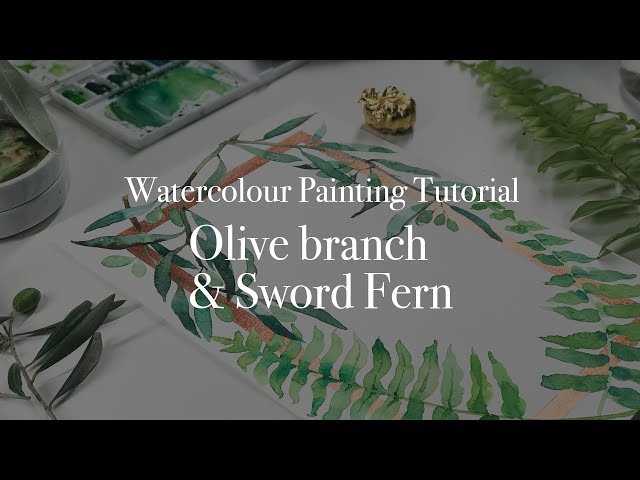The advertisement for the watercolor painting class features a meticulously arranged white table set against a jet black background, accentuating the art supplies and painting at its center. Dominating the table is a large piece of watercolor paper showcasing a detailed painting of olive branches, replete with lush, green leaves. Supporting this painting is a small wooden trellis, emphasizing the natural theme. Surrounding the artwork, to the left, lies an actual olive branch and a white flower, and to the right, a fern. Above the painting sits a small planter nurturing a live olive plant, adding to the verdant display. Additionally, on the upper left side of the table, there is a paint mixing tray spotted with various shades of green. White text prominently runs across the face of the image, declaring "Watercolor Painting Tutorial, Olive Branch, and Sword Fern," inviting viewers to engage with the class and immerse themselves in the art of watercolor painting.